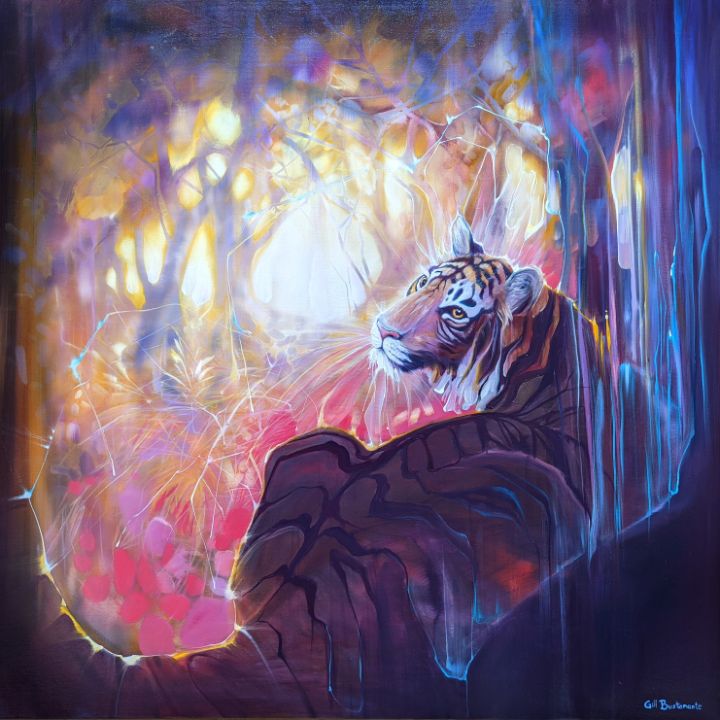This mesmerizing artwork features a tiger painted in a watercolor style, seamlessly blending mystical and fairy-tale elements. The tiger, with its characteristic black stripes, white around its eyes, and golden pupils, is depicted sitting and gazing over its shoulder. While its tail is not fully visible, it appears to curl around the lower left side of the image. The tiger’s orange and white face with intricate stripes adds a striking contrast against the dreamy, pastel hues of the background. The scene unfolds in what appears to be an enchanted jungle or forest, with lush trees depicted in shades of pink, purple, and blue.

The background further enhances the mystical atmosphere, evolving from dark shades at the border to lighter tones towards the center, creating a captivating depth. The forest-like setting is interspersed with bluish dripping effects and a central white focal area, making the tiger the undeniable centerpiece. In the lower right corner, a signature can be seen, likely stating “Gill” followed by an indistinct “B,” adding to the artistic authenticity. The overall composition, with its shadowy and pastel coloring, gives an impression of peering into a magical realm from the mouth of a cavern.